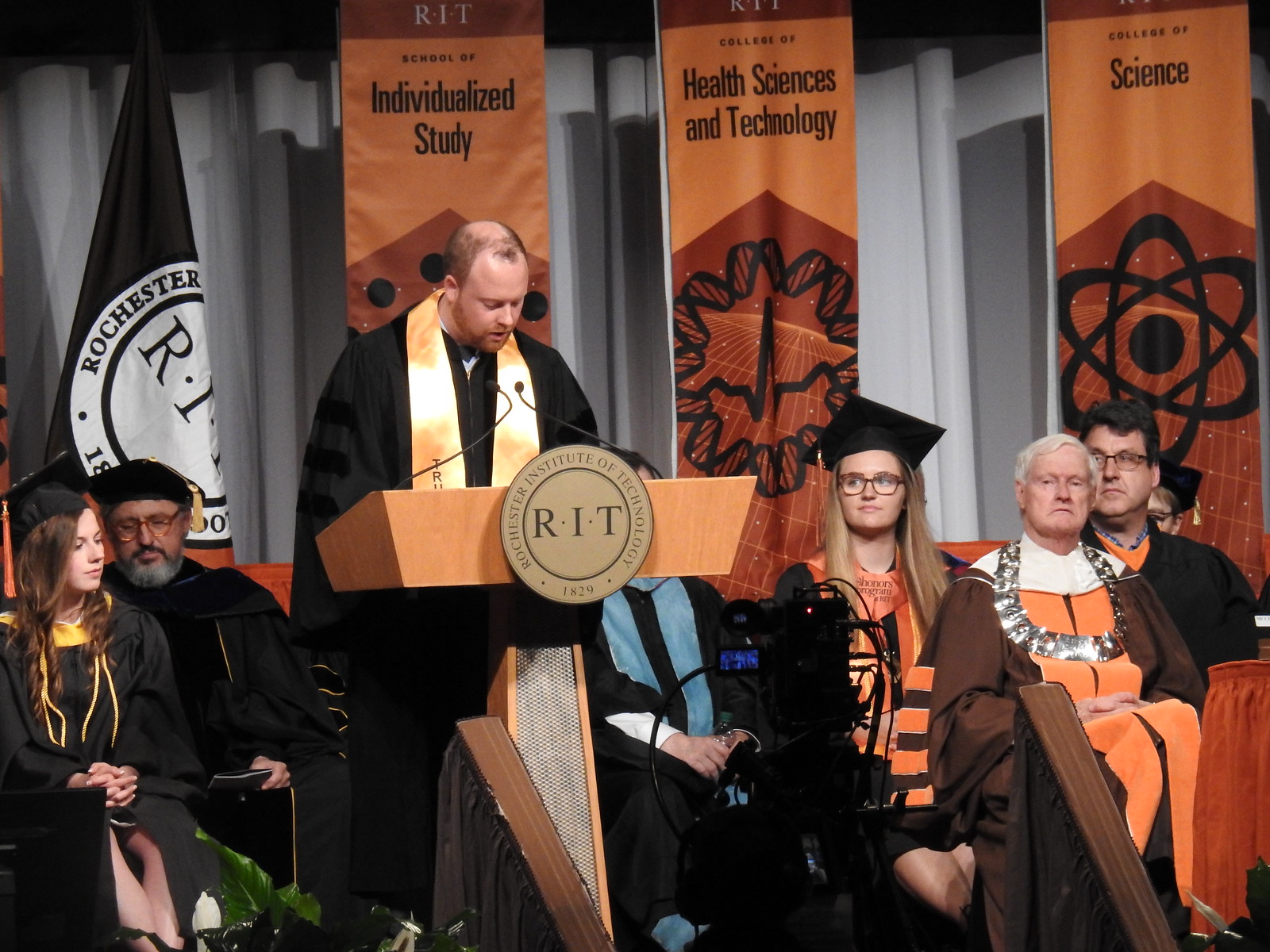The color photograph captures a commencement ceremony on a stage adorned with a white curtain and orange banners. The banners, with black lettering, read: “School of Individualized Study,” “College of Health Sciences and Technology,” and “College of Science.” At the center, a man with a red beard, wearing a black robe with a gold sash, stands at a wooden lectern bearing the emblem of the Rochester Institute of Technology (RIT), established in 1829. The lectern features two microphones. Surrounding him are individuals in graduation robes, some with caps and tassels. To his left, a girl and an older man are seated, and behind him, partially obscured, another person wears a blue sash. On his right sits a blonde woman with glasses, an older man with a metallic necklace, and another individual in black robes. Behind the group, a black flag with “Rochester RIT” text is visible. The scene is a detailed representation of a formal and celebratory academic event.